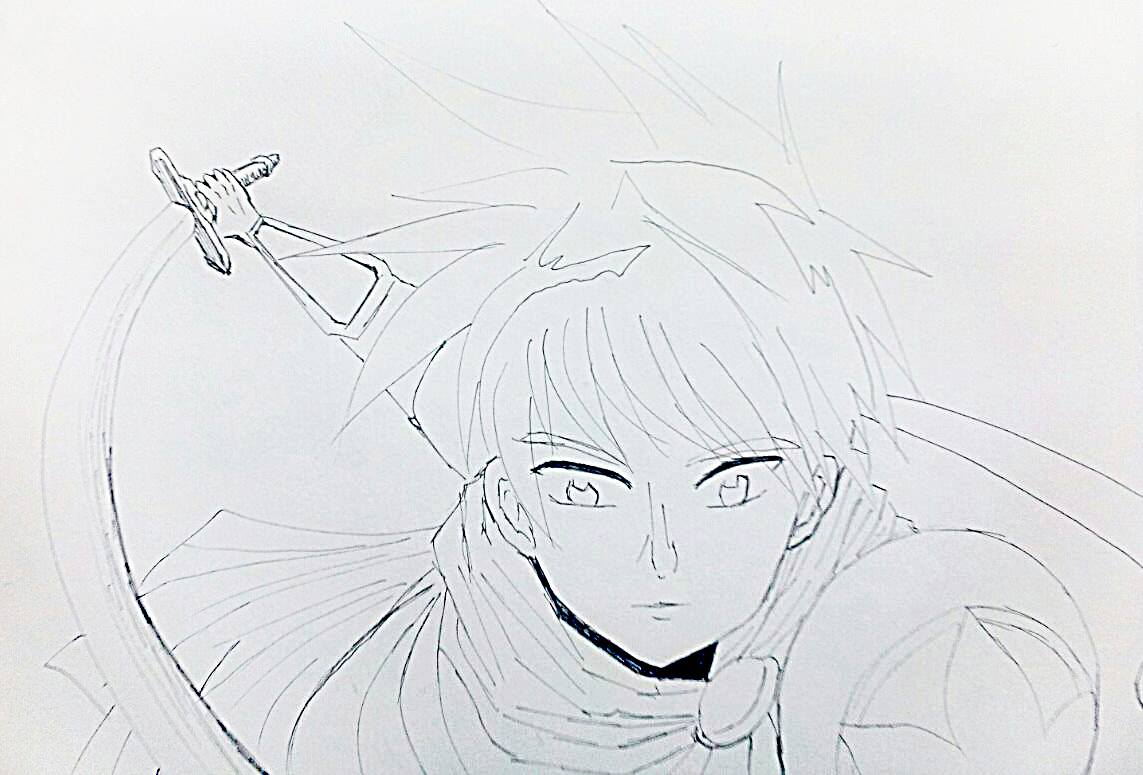The image is a highly detailed, black and white pen and ink illustration on a bluish-white background, featuring an anime-style warrior, possibly an elf. The drawing captures the warrior from the head down to the shoulders, facing forward as though addressing the viewer directly. The warrior has striking, spiky hair that is outlined in black ink, giving the impression of blond hair due to the uncolored white spaces within the lines. The warrior's facial features are finely rendered with big eyes that have heart-shaped irises, a thin nose, and delicate lips.

The character's right hand, on the viewer’s left side, holds a broad, curved sword resembling a scimitar, drawn back and held up behind their head, ready to swing forward. The warrior's left hand (on the viewer's right) brandishes a round, convex shield adorned with a leaf-like pattern. They are clad in shoulder armor, adding to their imposing and fantastical appearance. The overall scene hints at a moment of intense action, poised for battle.